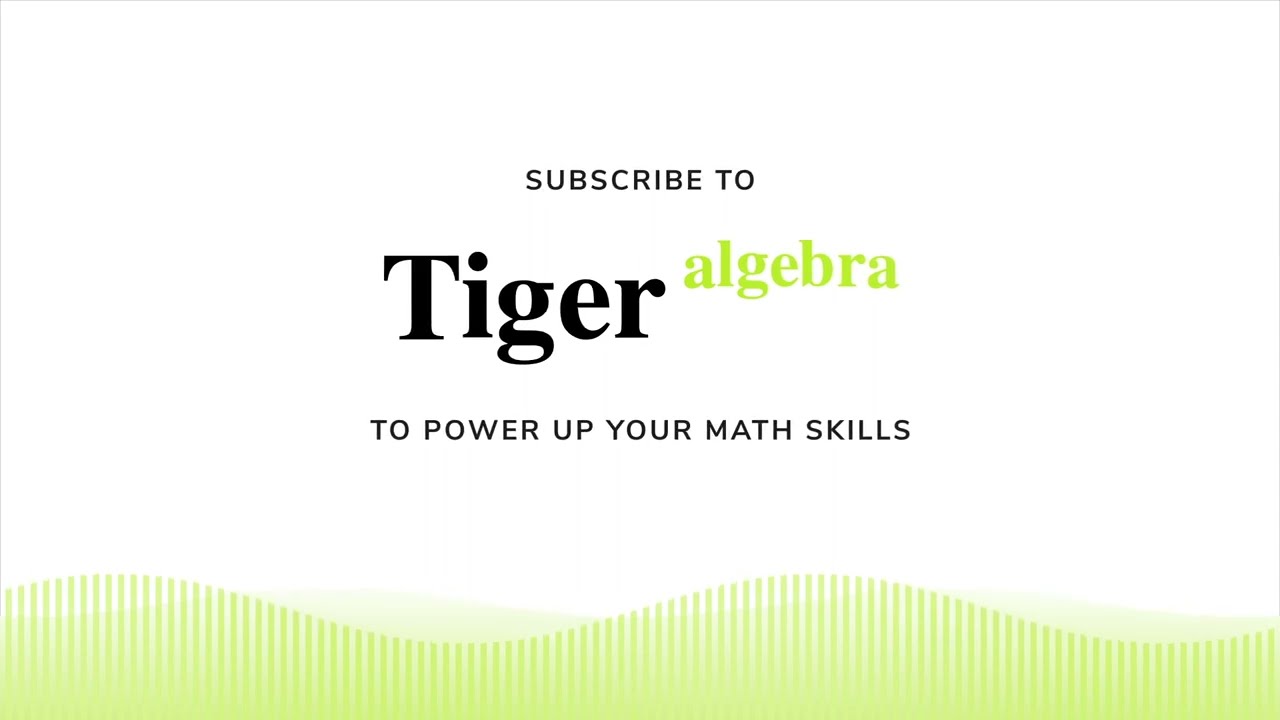The image is a promotional graphic designed to market a math service called Tiger Algebra. Set against a plain white background, the main text in the center of the screen reads, "Subscribe to Tiger Algebra to power up your math skills." The text "Tiger Algebra" is divided into two parts: "Tiger" is in large black font, while "algebra" is in lowercase lime green font, positioned near the top of the letter "R" in "Tiger." Below the text, a distinct green undulating line pattern resembling a waveform or hills spans the bottom of the graphic. The only colors present in the image are white, black, and shades of green, and the overall design suggests it is a piece of marketing material likely intended for use on a website or in a newsletter.